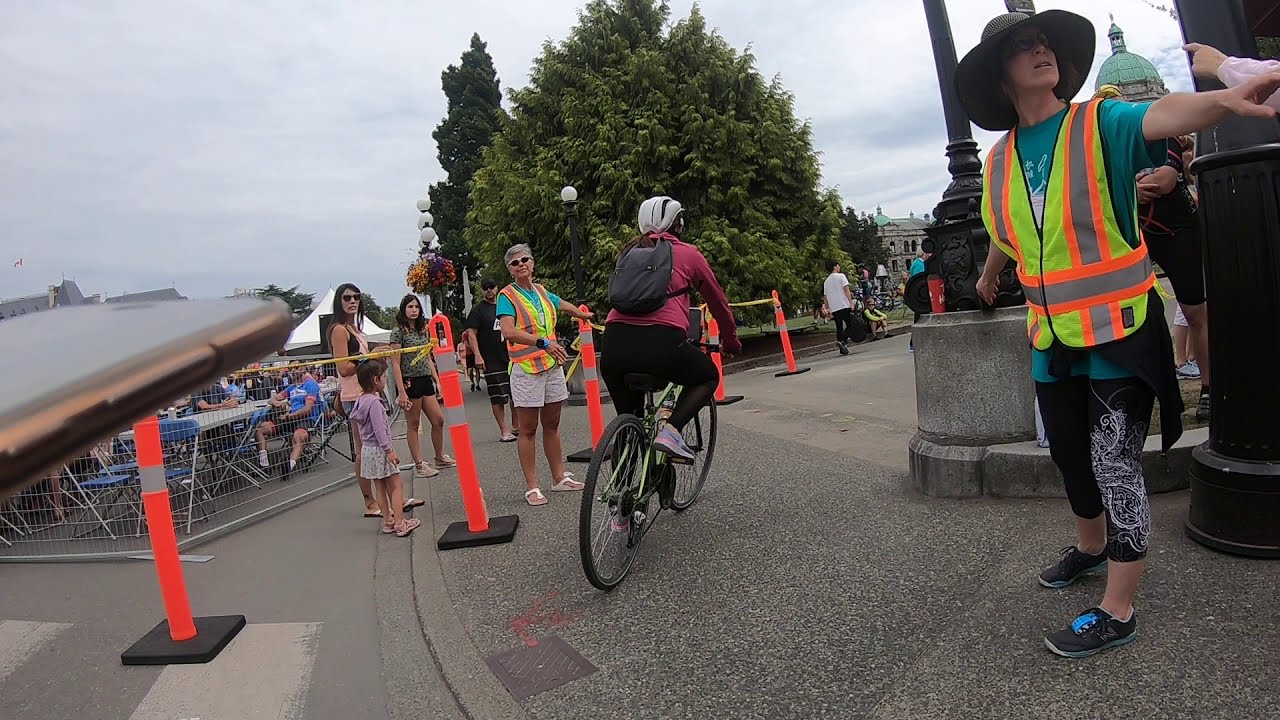In the center of the image, a man is riding a bicycle, seen from the back, wearing a white helmet, a black backpack, a red long-sleeved shirt, and black pants. Flanking him on both sides are two women directing traffic; each is dressed in neon yellow vests with orange and gray reflective stripes. The bike path is lined by a fence made of red poles with silver lines. Behind this fence, several people, including two women and a young girl, are standing and waiting, possibly cheering on the cyclists. Cones are set up along the path, and further back, a group of people are seated at tables, possibly eating and watching the event. The sky is cloudy, and the backdrop features some trees, lights, and buildings. The setting appears to be outdoors, in the middle of the day, at a bike racing event.